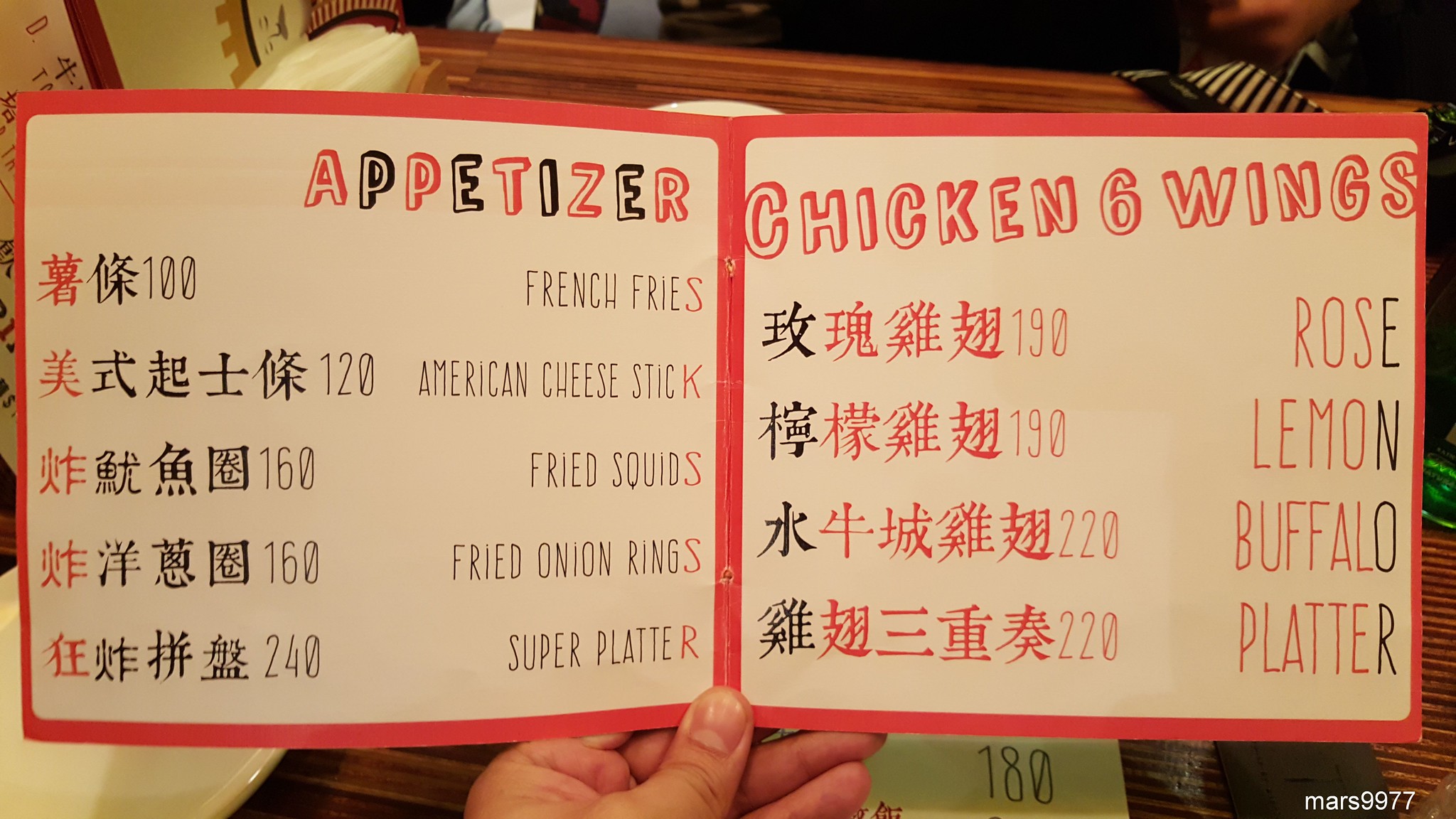An overhead view capture of a restaurant setting in a foreign country, featuring a detailed shot of a menu held by a person's hand. The restaurant interior is primarily composed of beige walls with strips of brown and tan, adorned with white and red symbols that contribute to the cultural ambiance. The table in the scene is brown, and the background, though slightly blurred, hints at an active dining environment.

The person's hand, visible from the bottom center of the image, is holding the menu, which is bordered in red. The menu itself is a mix of alternating black and red letters and symbols, presumably Chinese, listing various appetizers with their prices denoted alongside, such as '100' and '120'. The English translations include items like 'French fries' and 'American cheese sticks'. Adjacent to these listings, in white and red bubble letters, the menu offers 'Chicken six wings', again with translations and prices in both symbols and English. Toward the bottom of the menu, there's a notation in white that reads 'Mars 9977'.